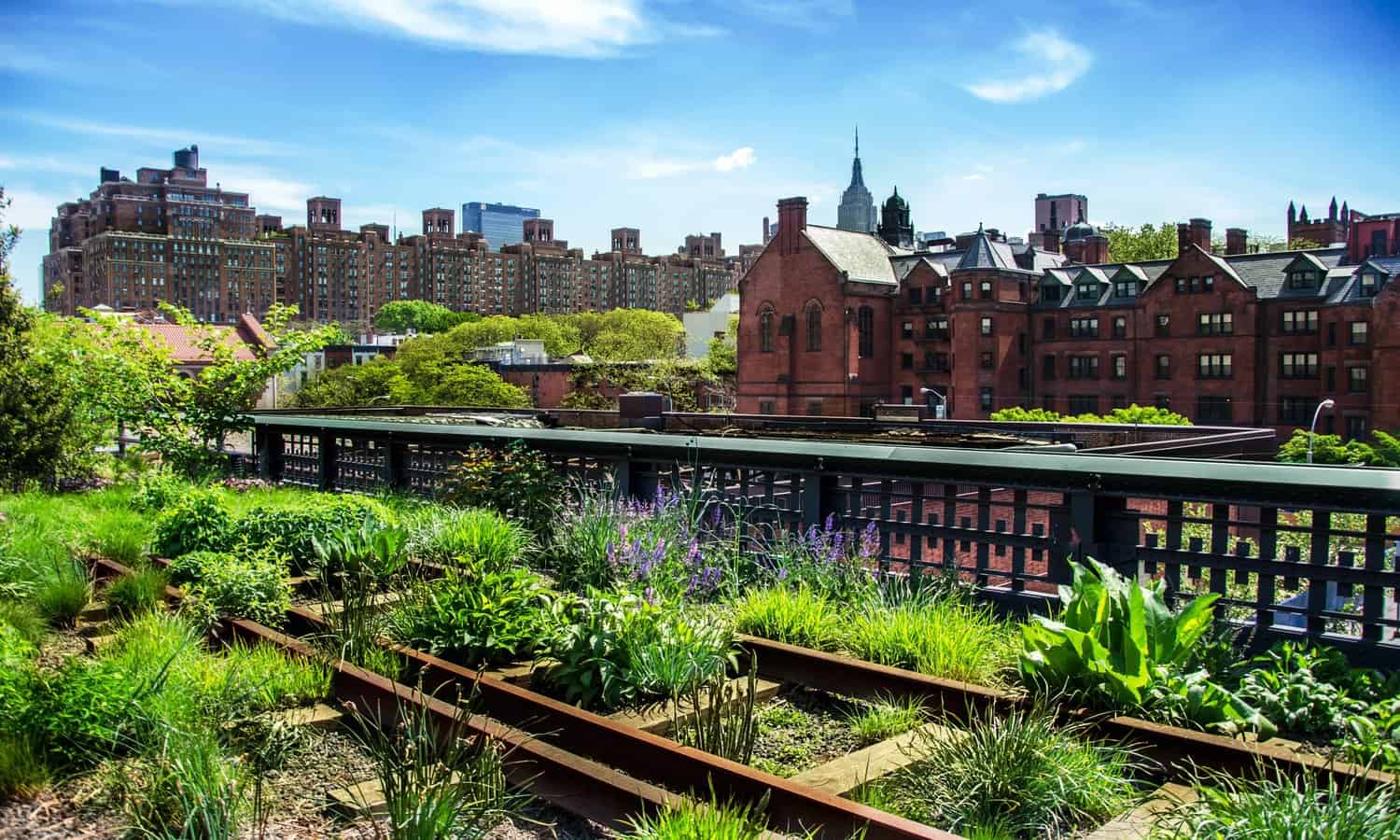In this picturesque scene of a quaint English town, a panorama unfolds with historical brick buildings standing shoulder to shoulder, exuding timeless charm. Dominating the background, a majestic steeple reaches skyward, a striking focal point against a serene canvas of clear blue sky dotted with fluffy white clouds. Below, a railway track, elevated on a grassy embankment, stretches languidly through the landscape. The track's iron rails, tinged with the red-brown hue of rust, hint at years of weathering. Paralleling the tracks is a long, vintage railway station, its facade punctuated by a continuous line of windows, evoking a sense of bygone journeys and the romance of train travel. Lush green grass frames the scene, thriving along the tracks and adding a touch of natural beauty to this charming townscape.